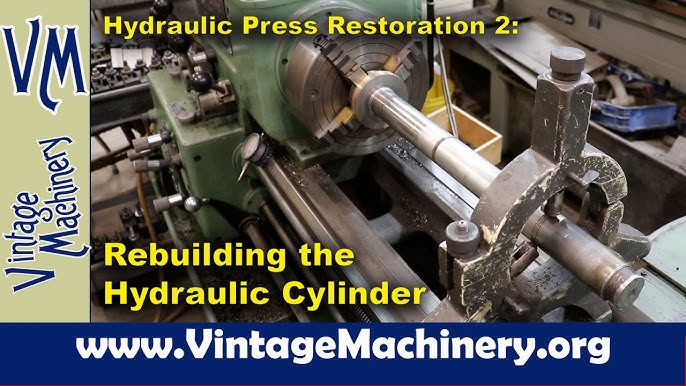This image is a detailed promotional poster for an instructional video or series on vintage machinery restoration. Dominating the upper left corner are the initials "VM" with "Vintage Machinery" beneath it, both set against a beige background. The main caption reads "Hydraulic Press Restoration 2: Rebuilding the Hydraulic Cylinder" in prominent yellow lettering. At the bottom, a blue banner with white text directs viewers to www.vintagemachinery.org. The central photo features a metal lathe holding a possibly worn hydraulic cylinder shaft, situated in a well-used yet functional machine shop. The hydraulic cylinder itself has a green base with black knobs and a silver-colored body, indicating it might be undergoing restoration. Overall, this poster provides comprehensive details about a vintage machinery restoration project, likely aiming to attract enthusiasts and professionals interested in hydraulic press repair and maintenance.